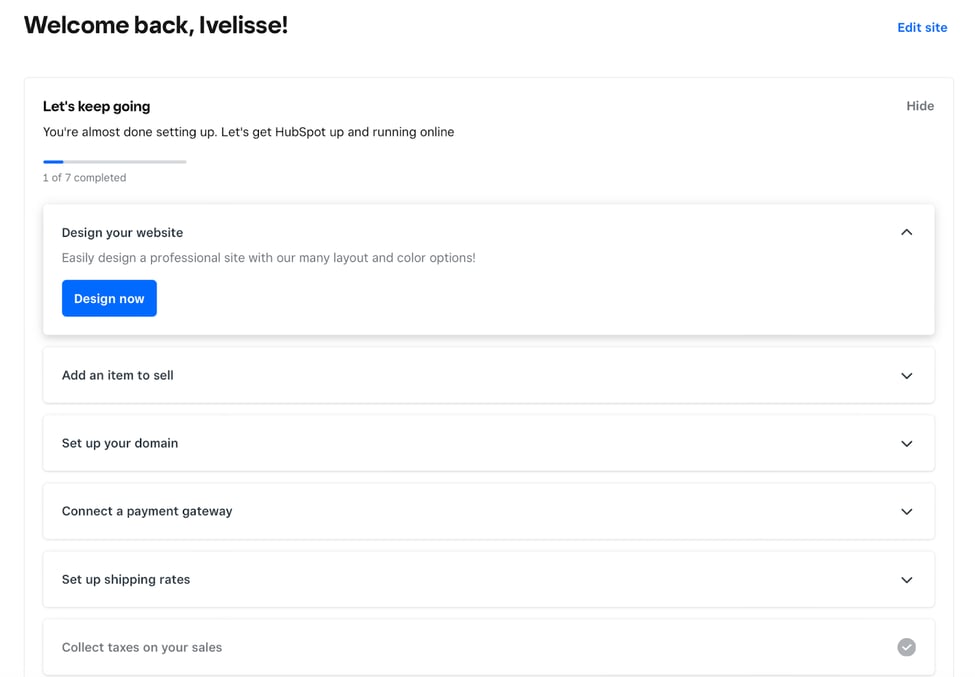The webpage displayed is rudimentary and simplistic, predominantly featuring a clean white background. The layout includes small boxes with sparse black text scattered throughout. At the top, in bold black text, it reads, “Welcome back, IVELISSE, I'm Leslie.” On the right side, there is hyperlinked text that says, “Edit Site.”

Just below, there is a white rectangular section bordered slightly in gray. Inside this box, bold black text proclaims, “Let's keep going.” Below this, regular black text states, “You've almost done setting up. Let's get HubSpot up and running online,” indicating that one of seven steps has been completed.

Subsequently, the next section appears selected. Bold text reads, “Design your website,” accompanied by gray text which says, “Easily design a professional site with our many layout and color options.” A dark blue clickable button with white text labeled “Design Now” is prominently displayed, and on its right side, an upward-pointing arrow adds emphasis.

Following this, several other rectangles with black text and down arrows are listed sequentially: “Add an item to sell,” “Set up your domain,” “Connect a payment gateway,” and “Set up shipping rates.” The last rectangle stands out with gray text indicating, “Collect taxes on your sales,” and instead of a down arrow, it features a dark gray circle with a white checkmark inside.